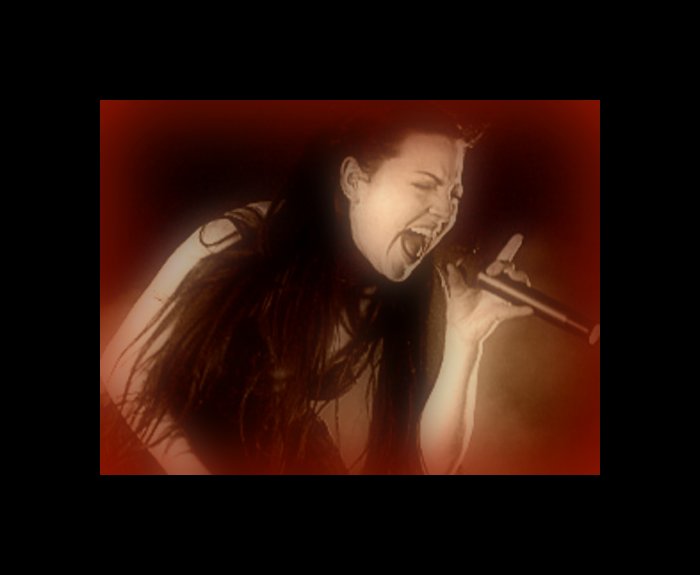This square, black-and-white photograph captures a powerful moment of a woman passionately singing, most likely during a concert. The image is framed by a thick black border, within which the photo itself has an intriguing ombre effect, transitioning from black to a reddish hue around the edges. The picture appears slightly blurry, with the center blown out in a grayish tone.

The woman is captured from a side angle, almost in profile, with her right side more prominently visible. She is gripping a long, black microphone in her left hand, with her index finger pointed upwards and her thumb extended. Her mouth is wide open and her eyes are closed, emphasizing her emotional involvement in the performance. She has long, black hair that obscures much of her outfit, but her visible biceps and forearms, along with the apparent sleeveless design, suggest she is wearing a black tank top or sleeveless shirt. Her facial features are distinctly clear, indicating she is of Caucasian descent.